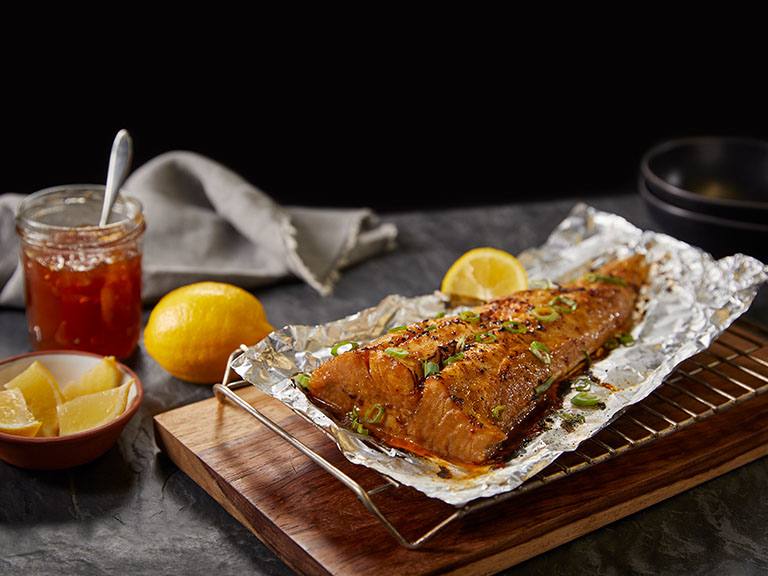The photograph showcases a delectable roasted fish fillet, its brown, crispy skin resting atop a rectangular sheet of aluminum foil. The foil catches a pool of savory sauce and oil beneath, capturing the richness of the dish. Sprinkled atop the fish are slices of green onions or chives, adding a splash of vibrant color. Nestled beside the fish on the foil is a fresh lemon wedge, ready to be squeezed for an added zing.

The aluminum foil sits on a slightly elevated steel cooling rack, which is itself placed on a rectangular wooden platter, creating a rustic presentation. This setup is arranged on a flat table draped in a black tablecloth, providing a stark contrast to the dish. To the left of the platter, there's a bowl filled with additional lemon wedges and a whole lemon, alongside a jar of honey, complete with a silver spoon. In the background, a couple of black bowls and a gray handkerchief are faintly visible, all against a completely black backdrop. The scene is perfectly lit, emphasizing the textures and colors, making the roasted fish fillet look incredibly appetizing.